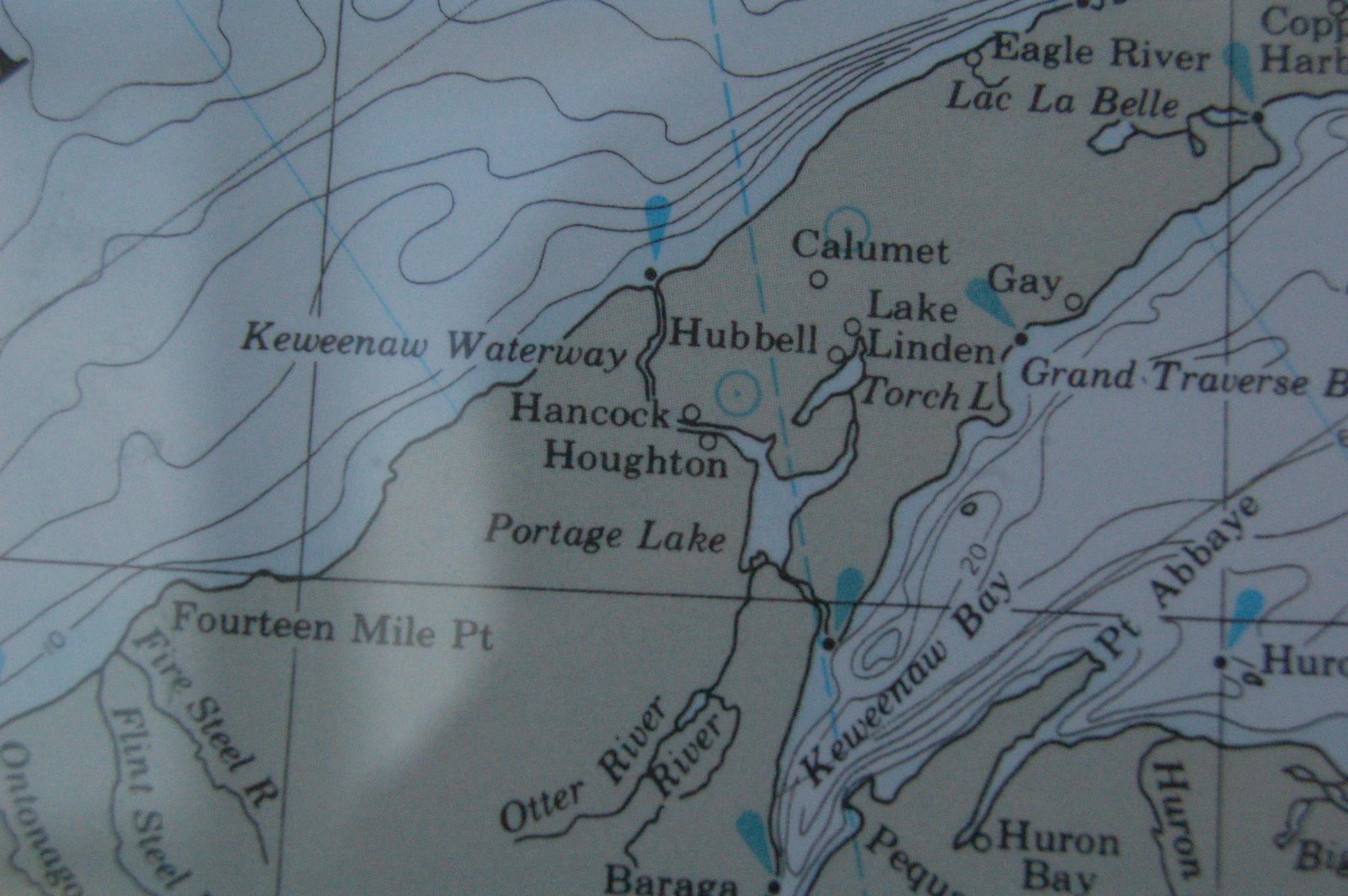This image captures a close-up photograph of a topographical map, showcasing a detailed representation of both land and water areas. The land is depicted in brown, while the water sections are shaded in light blue, with contour lines indicating depth. A grid pattern overlays the entire map, adding to its precise geographical detailing. In the center of the map, prominent landmasses are visible, blending seamlessly into numerous blue lakes and bays on the right side. The photograph also reveals the shadow of the photographer cast over the map, further emphasizing the close-up nature of the shot. Various place names are labeled throughout, including Eagle River, Lac LaBelle, Calumet, Lake Linden, Hubble, Keweenaw Waterway, Hancock, Houghton, Portage Lake, Otter River, 14 Mile Point, Firesteel River, Flintsteel, Pointe Abbey, Huron Bay, and Grand Traverse. Some names appear partially cut off, such as Ontonaga. Additionally, several oblong blue teardrop shapes are scattered across the map, though they remain unidentified. The combination of these details provides a rich and comprehensive view of the region depicted in the topographical map.